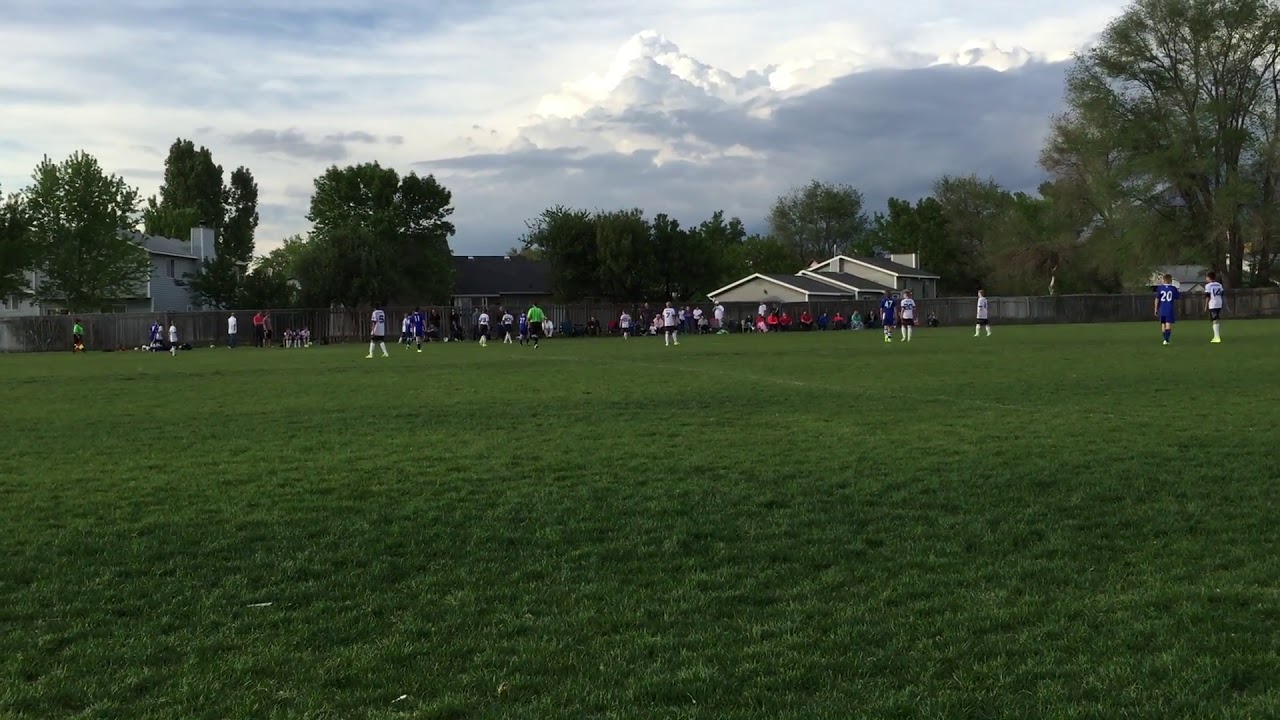The image captures an expansive, well-maintained grassy field under a somewhat overcast sky with patches of blue peeking through. In the middle distance, there are two sports teams assembled, identifiable by their uniforms: one team in blue jerseys, the other in white jerseys with black shorts, and a referee in a lime green shirt with stripes and black bottoms. The players bear numbered jerseys, suggesting they're engaged in an organized game, although the exact sport is not discernible. Behind the players, a row of spectators stands near a privacy fence that spans the width of the image. Beyond this fence, a subdivision with various houses and interspersed trees creates a backdrop. The scene is framed by a large tree on the upper right side and the sky, filled with both dense and wispy clouds that lend a dramatic, almost mountainous quality to the horizon.